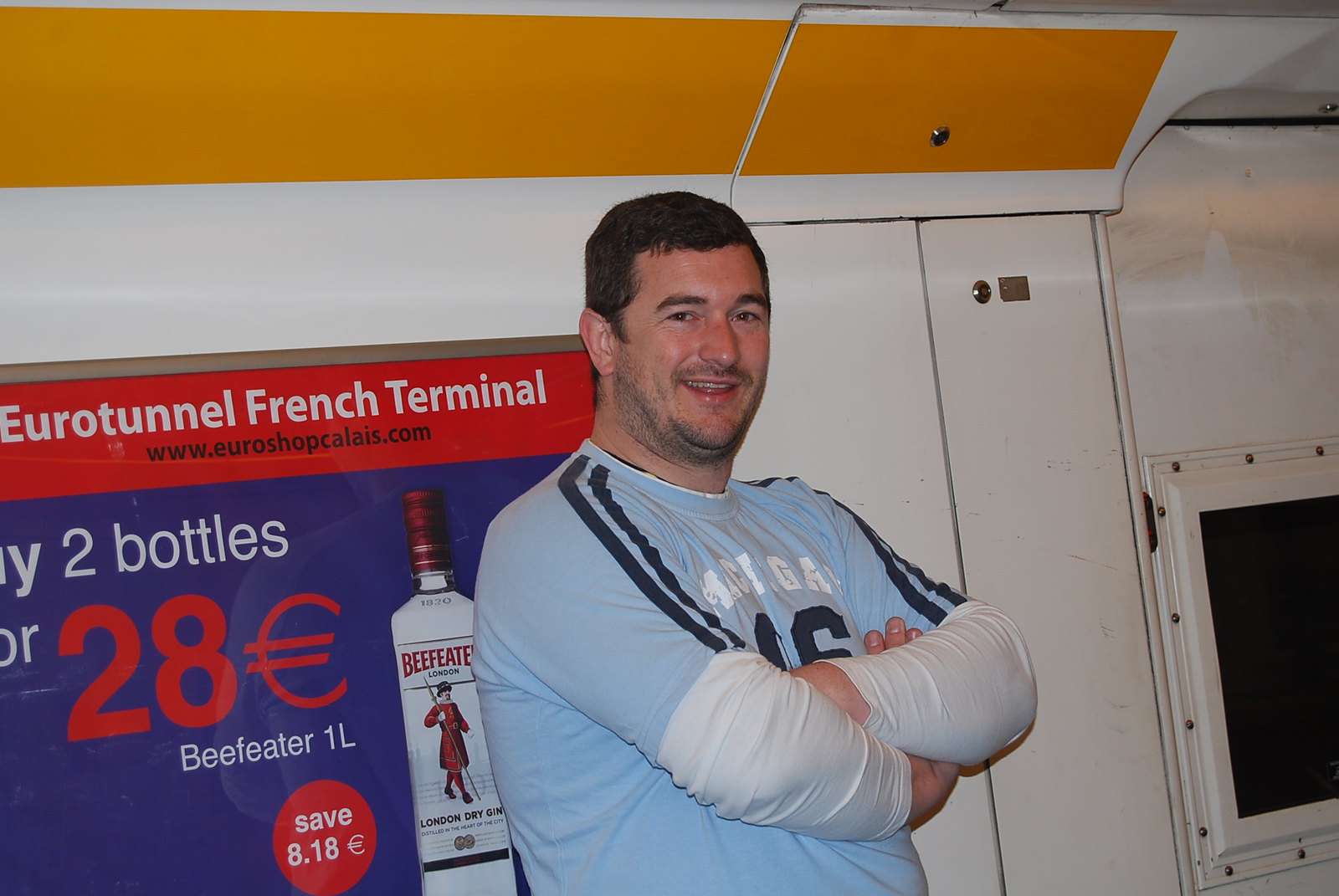The photograph is of a Caucasian man in his 30s, standing inside what appears to be a train compartment. He has dark short-cropped hair, dark eyebrows, and a stubbly mustache and beard, with fair skin. The man is smiling and facing the camera at a three-quarter angle to the right, with his arms crossed in front of his chest. He is wearing a light blue soccer t-shirt featuring dark blue stripes over the shoulders and white lettering across the front, which is partially obscured by his arms. Underneath the t-shirt, he has on a long-sleeve white shirt that covers his elbows and forearms. The photograph cuts off at his waist, so the rest of his attire is not visible.

In the background, the white interior walls of the train compartment are visible, along with overhead orange cabins or cabinets for storing gear. To the right side of the image, there's a white wall with a black square, likely a window. On the left side behind the man is a silver-framed horizontal banner advertisement with a blue background and an orange top border. The advertisement reads "Eurotunnel French Terminal," and below this, in black text, it reads "www.euroshopcalais.com." Featured prominently on the blue background of the advertisement is an image of a Beefeater bottle, a white bottle with a red cap and a red label featuring the word "Beefeater" over an image of a British soldier. To the left of this image, partially visible text reads "two bottles," and below that, bright orange numerals "28 €" followed by "Beefeater 1L" in white text, indicating a one-liter bottle. An orange circle with white text below this reads, "save 8.18 €." The man, seemingly enjoying the moment, is looking directly at the camera, providing a friendly and spontaneous vibe to the photograph.